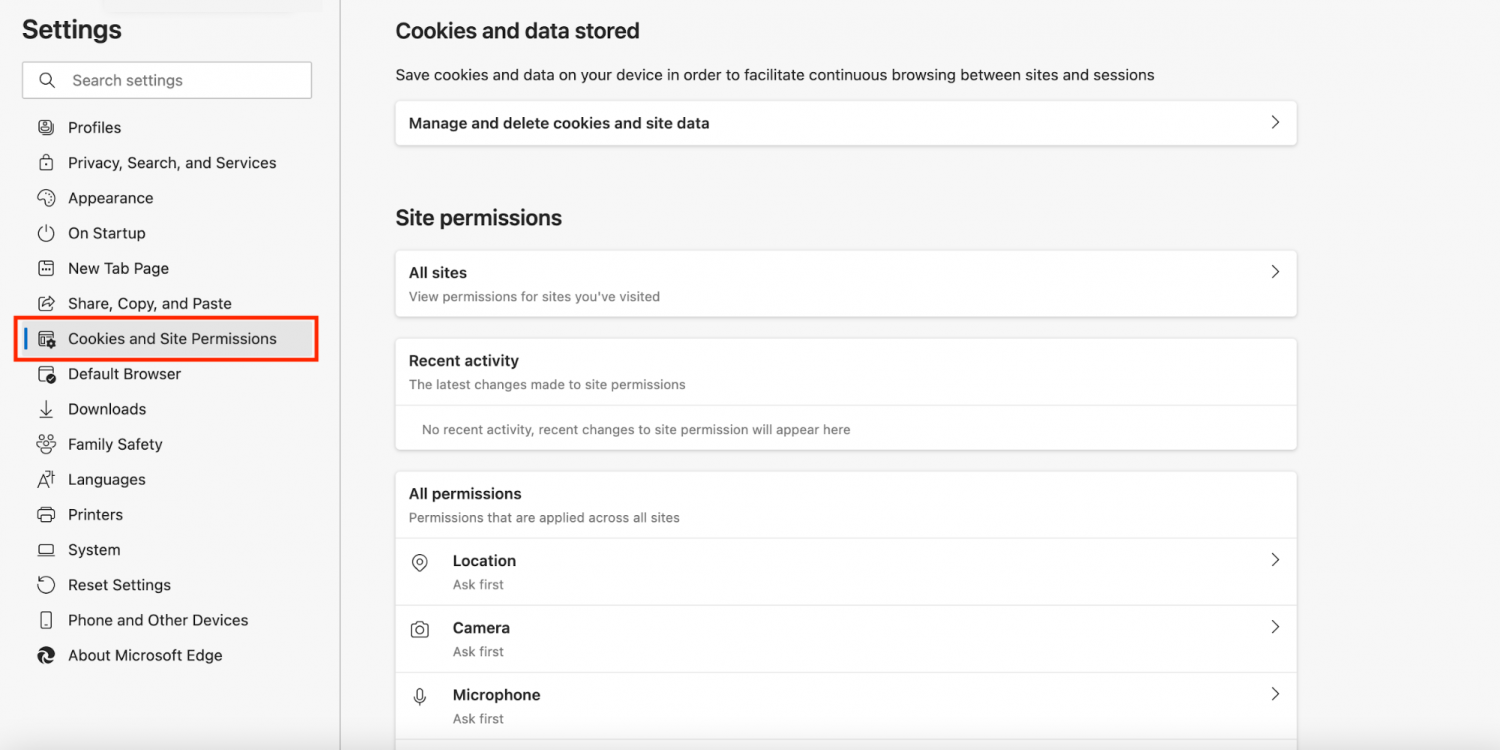The image displays the settings menu on a Microsoft device, showcasing a minimalist black and white theme. On the left-hand side, the word "Settings" is prominently displayed in black letters. Beneath it, there is a white search bar, outlined in gray, containing placeholder text that reads "Search settings" alongside a magnifying glass icon.

Following this, a vertical list of settings categories is presented in black letters with small corresponding icons, each separated by even spacing. These categories include:

- Profiles
- Privacy, Search, and Services
- Appearance
- On Startup
- New Tab Page
- Share, Copy, and Paste
- Cookies and Site Permissions (highlighted by a thick red border and a blue line next to its icon)
- Default Browser
- Downloads
- Family Safety
- Languages
- Printers
- System
- Reset Settings
- Phone and Other Devices
- About Microsoft Edge

To the right, in a larger section of the menu, "Cookies and data stored" is emphasized in bold black letters. Below this header, a brief description explains the function: "Save cookies and data on your device in order to facilitate continuous browsing between sites and sessions. Manage and delete cookies and site data."

Further down, the "Site Permissions" section is introduced, with options to view permissions for each site visited and recent activity logs. Currently, there is no recent activity noted with the placeholder: "Recent changes to site permissions will appear here." Finally, the "All Permissions" subsection lists various permissions that apply across all sites, with options for location, camera, and microphone, each labeled with the directive "Ask first."